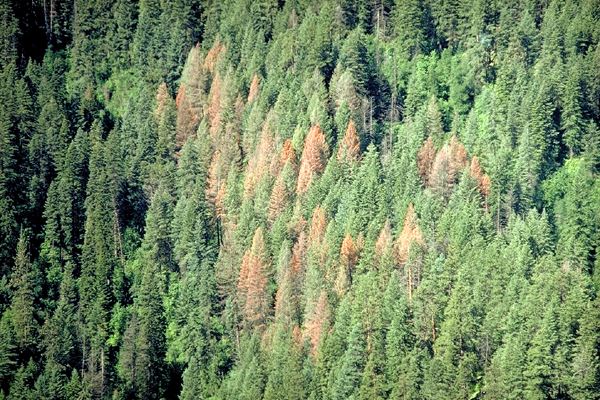This color aerial photograph, taken from a drone or helicopter, showcases a dense evergreen forest, likely consisting of fir, cedar, or pine trees, captured in a three by two aspect ratio. The forest canopy features a dynamic spread of green hues interspersed with areas of rust, orange, yellow, and brown. The trees on the left side appear darker and more sparsely distributed, potentially due to the shading from a hillside or mountain slope. As the focus shifts towards the center and right side, the trees are densely packed, with some displaying signs of natural decay or environmental stress, such as blight or seasonal color change. These affected trees are sporadically spread, creating a patchwork of vibrant green alongside browning and dying trees. The image, devoid of any text, presents a striking visual of nature's varied palette and the contrasting health of the forest ecosystem.